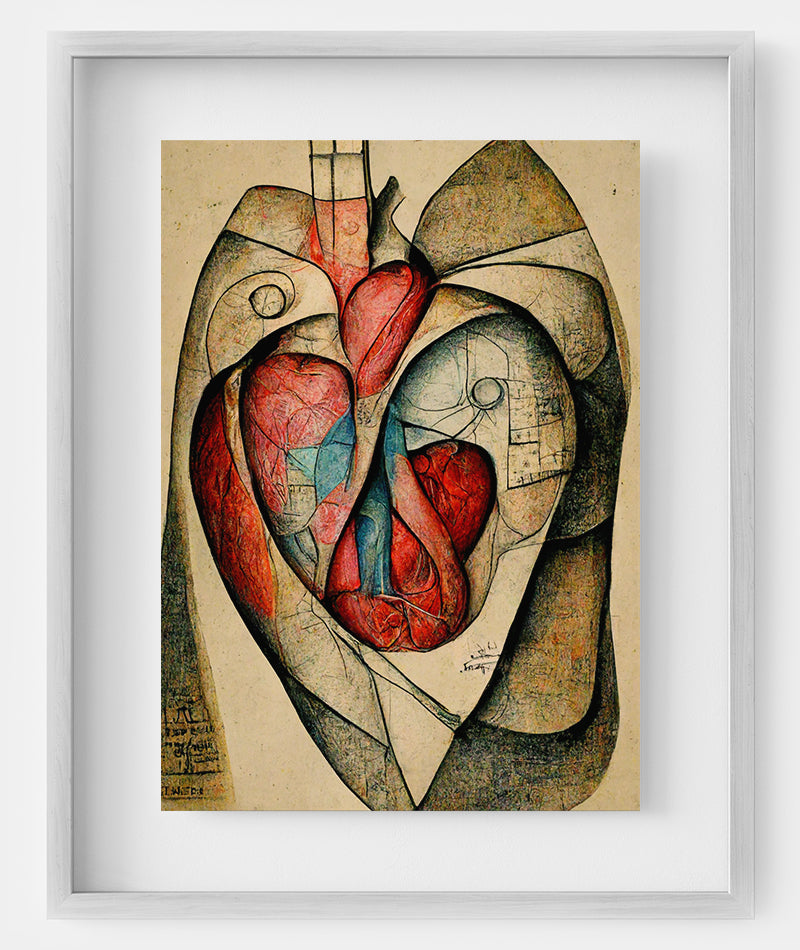This is a framed artwork featuring an abstract, stylized rendering of an anatomical human heart. The piece is encased in a thin, grayish frame with a white mat border. The artwork's focal point is a heart-like shape with red and blue valves and several chambers, suggestive of an anatomical heart. Surrounding this central heart are abstract elements resembling folded paper layers in shades of white, off-white, and tan, with shading around the edges. These layers create an intricate texture around the heart shape, which also has a vaguely cartoonish heart outline integrating into its form. The background of the artwork is a sand color, adding a soft, muted contrast to the vibrant reds and blues. There is some unreadable writing in the bottom left corner of the piece, adding an additional layer of intrigue.